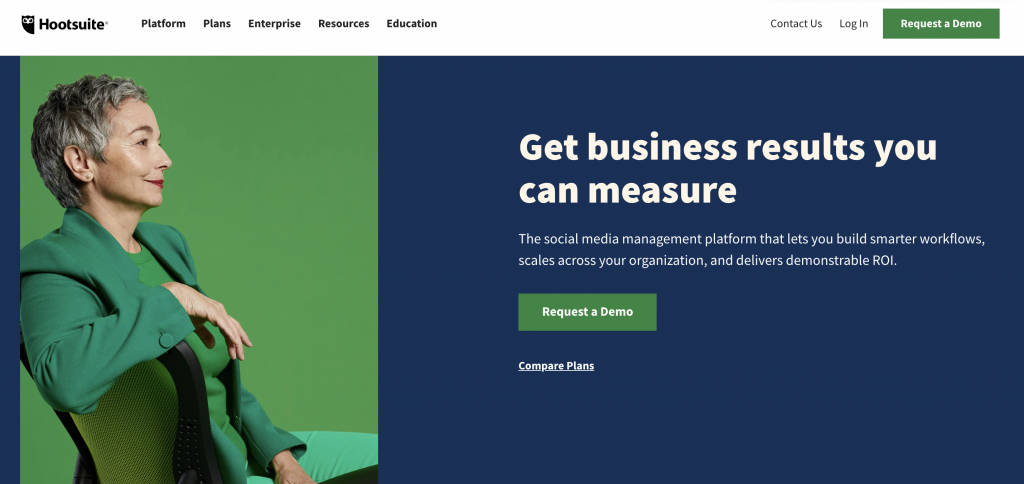The image illustrates a landing page for the website Hootsuite. Dominating the top left corner is the brand's logo, consisting of the name "Hootsuite" accompanied by a cartoon owl. Adjacent to the logo, a white header hosts several navigational buttons labeled Platforms, Plans, Enterprise, Resources, and Education. Positioned on the far right of this header are additional buttons for Contact Us, Login, and a prominent green button labeled Request a Demo.

Below the header section, the visual splits into two contrasting sections. On the left, a woman dressed entirely in green is seated against a matching backdrop. She has short gray hair and dons a green suit jacket, green shirt, and green pants, all blending seamlessly with the green chair and background. To the right, a blue background carries bold white text stating, "Get Business Results You Can Measure," followed by a detailed description of the platform: "The social media management platform that lets you build smarter workflows, scales across your organization, and delivers demonstrable ROI." At the bottom of this text block, another green button invites users to Request a Demo.